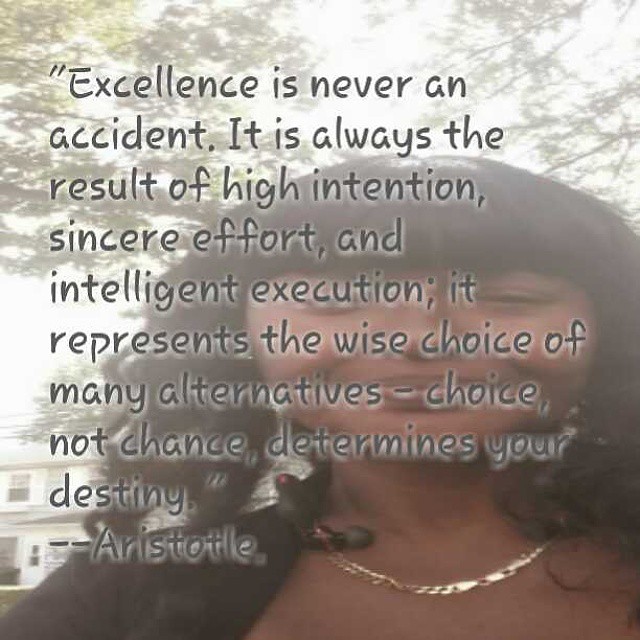This image, likely intended for a social media post, features a motivational quote superimposed over a blurry, soft-finish photograph of a smiling woman. She has long, wavy black hair cascading past her shoulders and is accessorized with a gold chain necklace. Her eyes are softly closed, adding to the serene expression. The background reveals the tops of treetops and, on the left-hand side, a partial view of a two-story house with windows and shutters. The inspirational quote, displayed in a casual font, reads: "Excellence is never an accident. It is always the result of high intention, sincere effort, and intelligent execution. It represents the wise choice of many alternatives. Choice, not chance, determines your destiny." This quote is attributed to Aristotle and is enclosed in parentheses, followed by two dashes and Aristotle’s name.